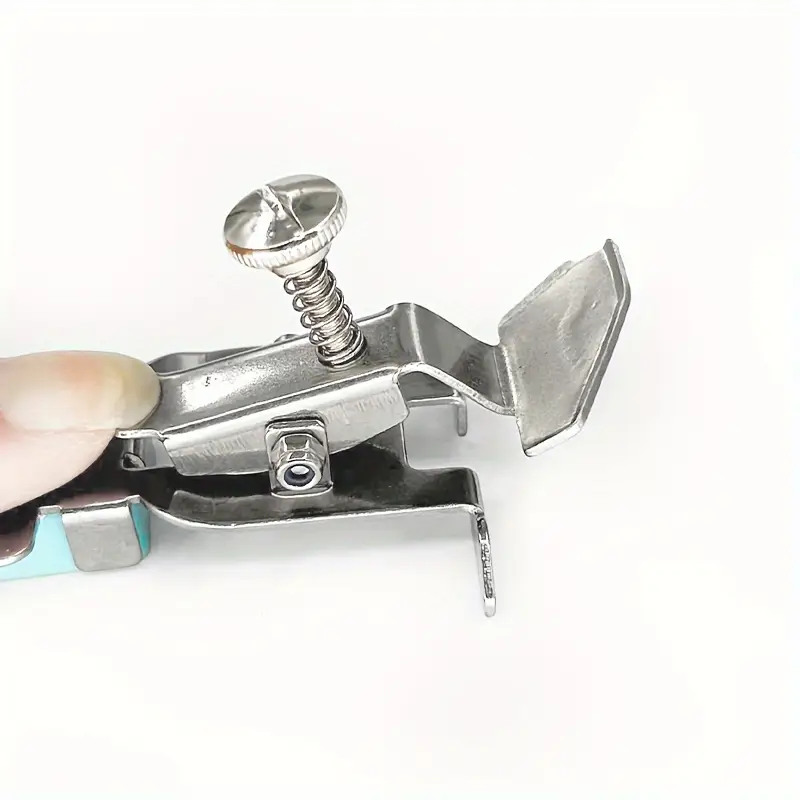The photograph showcases a small, shiny metal clamp, primarily silver in color, set against a white backdrop with no text or markings. To the left, a pale, Caucasian fingertip with a long, neatly trimmed nail, possibly from a female, is pressing down on the back portion of the clamp, suggesting it is spring-loaded and easy to manipulate. The clamp itself features a circular top with a cutout designed for a flat-top screwdriver, connected to a post with a screw and spring mechanism visible at the upper section. The structure then slopes downward and leads into a large, angular metal piece resembling a rectangle with cut angles and an additional downward slope. Adding a touch of color, a blue design accents the bottom section of the clamp. Despite the detailed visual elements, the exact function of the tool remains unclear, evoking curiosity about its practical use.